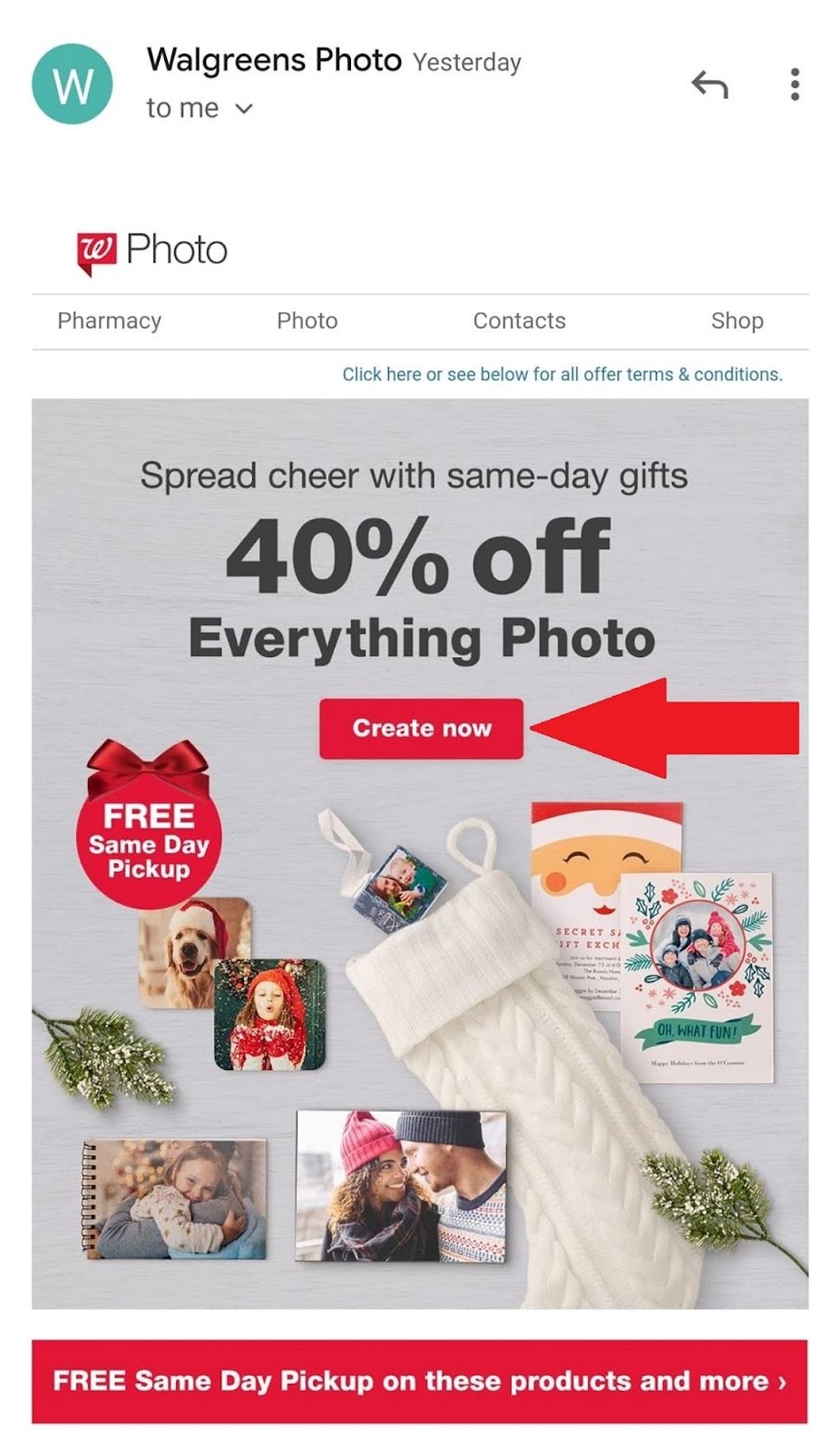The image is a promotional graphic for Walgreens, embedded in an email sent to customers. The top of the graphic shows a banner with the Walgreens logo and navigation options including "Pharmacy," "Photo," "Contacts," and "Shop." Beneath this banner, a call-to-action text encourages users to "Click here to see below for all offers and terms." 

The main section of the poster displays a festive gray surface adorned with various Christmas-themed elements. Scattered across the surface are gift cards, little notebooks, sprigs of mistletoe, Christmas stockings, and colorful ornaments. Among these items, a highlighted message announces "Free same-day pickup on these products and more," directing users to an embedded link.

An eye-catching red button labeled "Create Now" is prominently displayed, offering "40% off everything, photo." An arrow points directly to this button, emphasizing its importance. The entire composition is designed to highlight holiday-themed products and Walgreens' photo services, emphasizing the convenience of free same-day pickup for personalized holiday gifts.